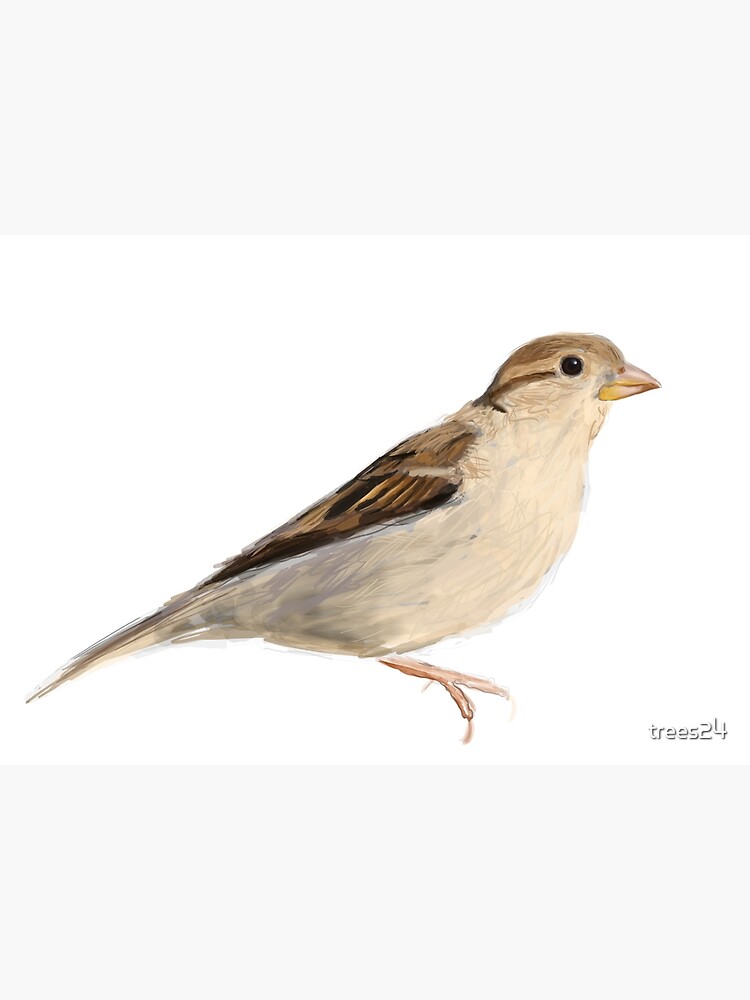A digital illustration depicts a bird, possibly resembling a sparrow, set against a white background bordered by light gray rectangles at the top and bottom. The bird is seen in profile, facing to the right. The bird's plumage showcases a gradient of earthy tones: its head and back feature darker browns, almost black in areas, while its underbelly transitions from a very light tan to a darker gray towards the tail. The wings and tail mirror the darker brown hues of the head. It sports a yellow beak and feet, which have a dull yellow to orange tint. A distinguishing dark streak runs from its black eye, further adding to the detailed coloration. Despite being a drawing, the bird is posed naturally, standing upright with no visible perch, centered in the larger white space.